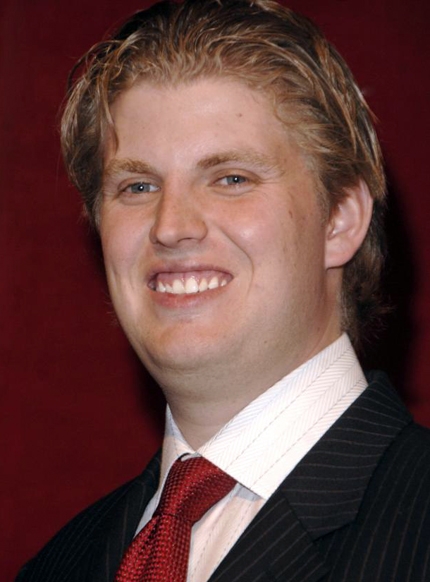A professionally taken photograph features a man in his thirties, who bears a resemblance to Donald Trump Jr. The individual has a fair complexion, clean-shaven face, and reddish blonde hair that is about two to three inches long, hanging slightly towards his eyes. His bushy eyebrows match the reddish blonde hue of his hair. He has a heavier build and is dressed formally, wearing a white collared shirt with subtle black pinstripes, a dark red tie, and a black jacket adorned with white pinstripes. The backdrop of the image is a deep red, felt-like material, suggesting a professional photography setting. The man is smiling directly at the camera, exuding a polished and approachable demeanor.